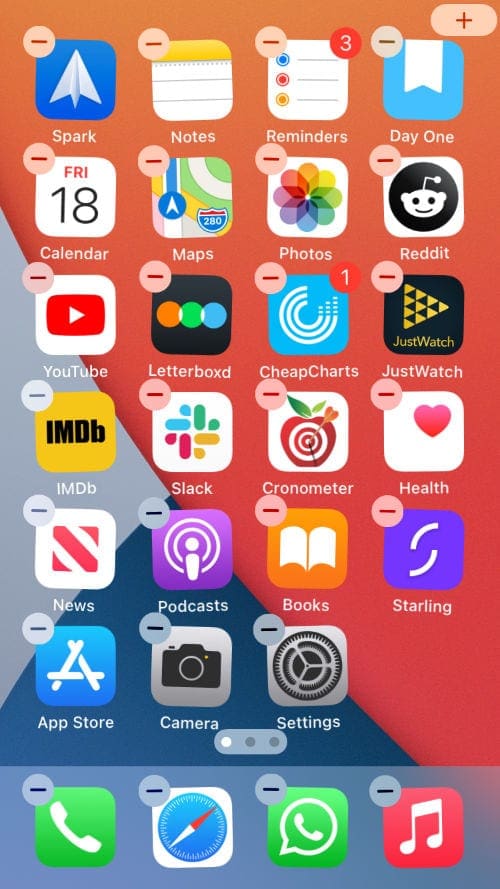The image depicts the home screen of a smartphone or iPod with a multi-colored background. The dominant hues are primarily orangish-pink, stretching diagonally from the right corner to the left corner, while the left side features a gray triangle and a dark blue triangle at the bottom, completing the vibrant background. At the bottom of the screen, a menu bar shows various app icons, each accompanied by a gray circle with a negative sign, indicating that the icons are in a deletable or movable state.

In this menu section, notable app icons include a white phone in a green circle, a navigation button, another phone icon enclosed in a circle, and a red rectangle with a white music note. The main display is densely populated with multiple icons, possibly representing various apps or connectivity features, arranged in a grid of four columns and five rows. All spaces are filled except for the bottom right corner, which remains empty.

Additionally, a pill-shaped button with three dots is visible at the bottom, signifying the total number of pages on the device. The first dot is white, indicating that this is the currently active page. Overall, the layout is symmetrical and evenly organized, providing a neat and visually pleasing arrangement of the home screen elements.